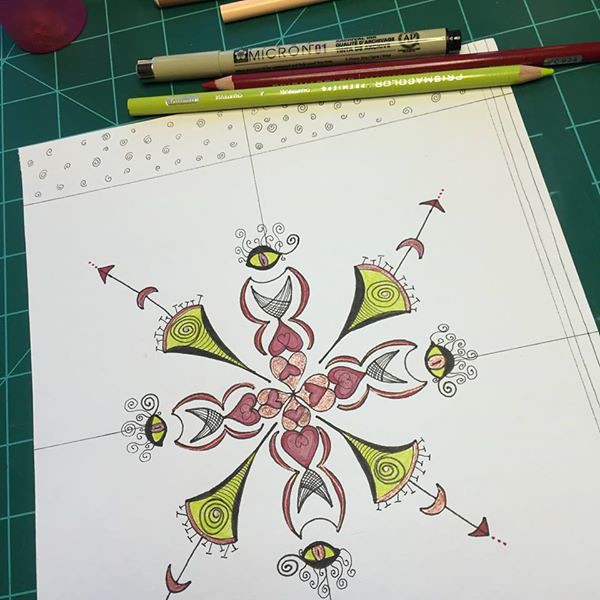This image features an intricately detailed contemporary drawing on off-white paper, laid atop a hunter green graph paper with white lines and boxes. The artwork is a highly symmetrical blend of abstract shapes and designs, rendered primarily in maroon (rust) and lime green colored pencils, which are visible at the top of the image along with a black marker. The drawing evokes a floral or snowflake-like pattern with a plus-shaped structure, featuring hearts and crescent shapes radiating from the center. The composition includes an eyeball with a black lid and a triangular shape with a sharp point. The upper border is decorated with petite designs, complementing the three vertical lines on the right side. Overall, the piece is an original, modern design executed with precision and creativity.